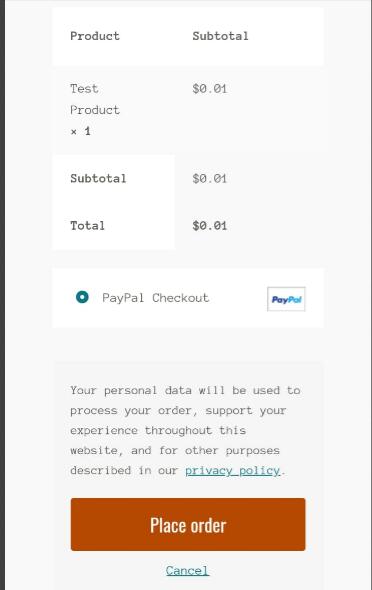This image depicts a digital receipt against a predominantly gray background. The receipt features a simple, uncluttered layout without any company name or logos at the top or bottom. The item listed is "Test Product," priced at $0.01, noted as "Test Product x1." The subtotal and total both reflect this amount, $0.01, and are housed within white boxes.

On the left-hand side of the receipt, there is a green illuminated circle. To the right, the PayPal logo is prominently displayed, signifying that PayPal checkout is available. Below this, there is a message indicating that personal data will be used to process the order, enhance the user experience on the website, and for other purposes as described in the privacy policy, which is highlighted in green and underlined.

At the bottom of the receipt, there's a large rust-colored button labeled "Place Order" in a tan font, followed by a smaller "Cancel" option written in blue with an underlining of the same color. The entire graphic is bordered on the left side by a thick black line and on the right side by a much thinner black line.